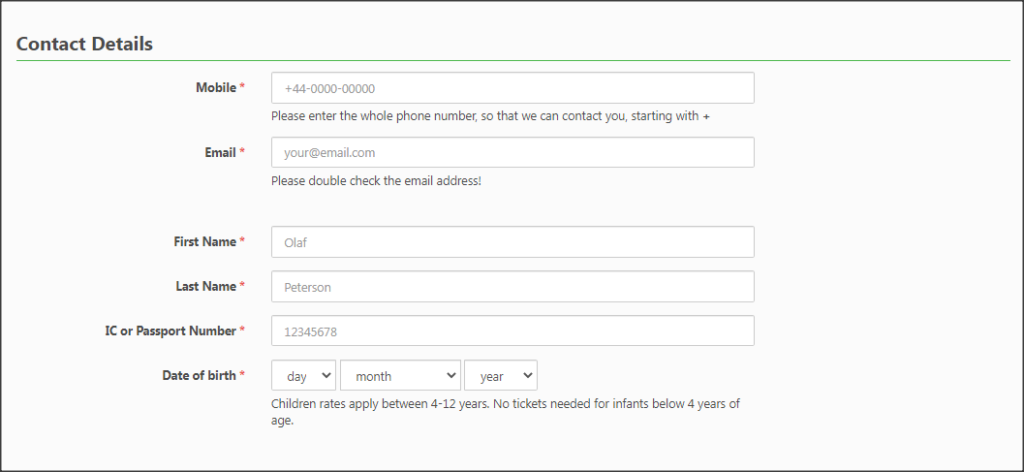The image depicts a form designed for collecting contact information, prominently located in the top left corner of the visual. The form is enclosed within a light gray to white box, bordered by a distinct gray line that sets it apart from the white background. At the top, a green line runs horizontally, acting as an underline to the title or header of the contact details section.

This structured form consists of multiple long, skinny rectangular fields where users can input their details. Each field is prefaced by a label with a red asterisk, indicating that the information is required. 

The first field, labeled "Mobile" and marked with an asterisk, comes with a clear instruction: "Please enter the whole phone number starting with '+', so that we can contact you." An example number featuring zeros is provided as a format guide. 

Beneath this, the "Email" field also bears a red asterisk and underscores the importance of accuracy with the note: "Please double-check the email address!" 

Following these, the form requests additional personal details, starting with the first name, exemplified by "Olaf," and the last name, exemplified by "Peterson," both of which are mandatory. Additionally, the form seeks the respondent's IC or passport number and date of birth, specifying the required format of day, month, and year.

This detailed design ensures clarity and precision, enhancing the ease of use while emphasizing the importance of accurate and complete submissions.